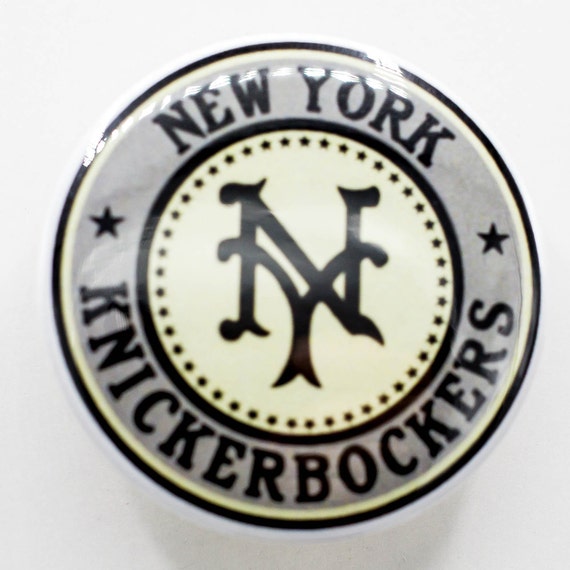This photograph captures an enamel lapel pin against a white background, possibly intended for online sale. The pin is circular, featuring a shiny, polished finish. The outermost part of the pin has a black outline. Just inside this outline is a ring of light blue or gray with the text "New York" at the top and "Knickerbockers" at the bottom. Between the words "New York" and "Knickerbockers" on either side are two black stars. Encircling the inner part of the pin, there is a series of small black stars embedded within a thick black border. At the heart of the pin, enclosed by yet another black circle, lies a cream-colored or ivory center. Inside this center, the letters "N" and "Y" are overlapped, styled similarly to the New York Yankees logo but distinctly unique. The N is overlaid atop the Y in a bold, black font. The overall color scheme of the pin includes shades of gray, cream, and black, with multiple concentric circles defining the design elements. The photograph, although slightly blurry, effectively highlights the detailed and intricate craftsmanship of the lapel pin.